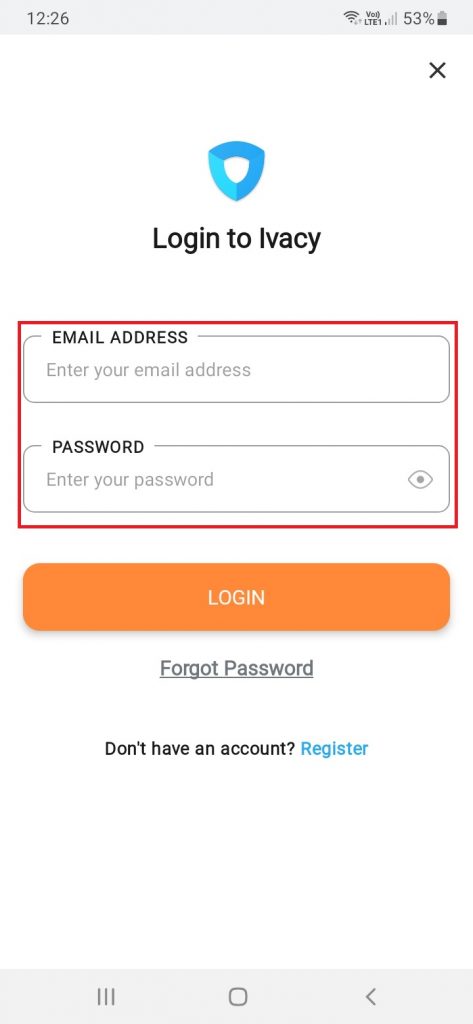This image is a detailed screenshot of a cell phone screen running the Android operating system, as indicated by the specific icons and layout. 

### Top Bar Details:
- **Time:** 12:26 (located at the top left).
- **Wi-Fi Status:** Full Wi-Fi bars (located at the top right).
- **Cellular Strength:** Displays LTE with only a single bar of cellular signal strength.
- **Battery Level:** The battery is at 53%.

### Bottom Bar Details:
- **Three Navigation Icons:** 
  - Icon 1: Three vertical bars (likely the app drawer or menu button).
  - Icon 2: A square with rounded edges (the recent apps button).
  - Icon 3: An arrow pointing to the left (the back button).

### Main Screen Focus:
- **App Login Interface:**
  - **Title:** "Log in to IVACY" displayed within a blue shield outlined by a white interior.
  - **Form Fields:** 
    - **Email Address:** A box to enter the email address.
    - **Password:** A box to enter the password, accompanied by a small eye icon to toggle password visibility.
  - **Action Buttons:**
    - **Orange Login Button:** A wide button labeled "Log in."
    - **Additional Links:** 
      - "Forgot password" for password recovery.
      - "Don't have an account? Register" for new users to create an account.

The screenshot clearly represents the login screen for the IVACY app, providing users with options to log in, recover forgotten passwords, or register a new account.